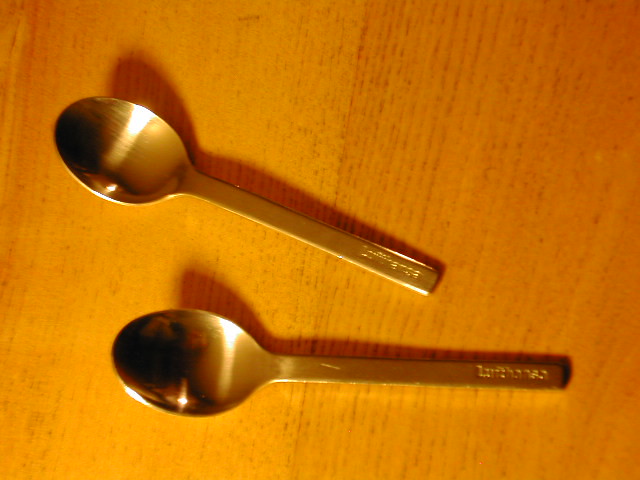This color photograph captures a top-down view of two silver spoons placed on a light brown wooden table, displaying intricate details. The table's wood grain runs vertically and features dark brown and light grayish-black streaks, adding texture to the scene. The spoons are arranged with the spoon bowls pointing to the left and handles to the right.

The bottom spoon lies perfectly horizontal, while the top spoon is slightly tilted, creating a subtle visual dynamic. Both spoons are short and slender, with rectangular handles and some barely visible etched writing at the handle tops. The spoon bowls reflect the ambient light, giving them a shiny appearance that introduces a warm, almost golden hue to their silver surface.

Shadows cast by the spoons add depth, with a notable shadow appearing on the bottom spoon that shows a partial reflection, possibly of the photographer. The overall scene is enhanced by the yellowish light source from the left, which amplifies the wood's color variance and adds a soft glow to the metal utensils. The image is serene and minimalistic, with no other objects in view, emphasizing the simple elegance of the spoons and the natural beauty of the wooden table.